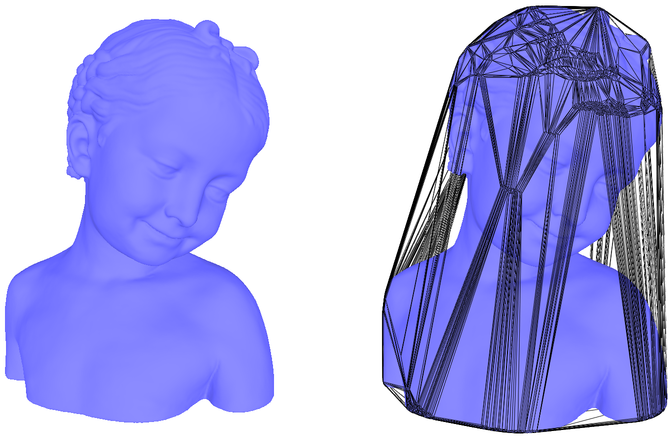In this detailed image, we see a side-by-side comparison of a 3D-rendered, purple bust of a young child, depicted from the chest up. Both busts are almost identical, showing the child with a slight grin, eyes closed, and head tilted slightly to one side. The child has wavy hair with a bow at the top. The sculpture is rendered with a smooth purple finish, making it difficult to distinguish fine details.

The left bust features the child with no additional adornments. On the right, the same bust is overlaid with a black, intricate, spider-web-like veil pattern that drapes over the entire head and chest. The pattern is denser at the top, thinning out with longer, straight lines toward the bottom and sides, creating an intricate and mysterious visual effect. This veil or pattern gives the right bust a distinctly different texture and appearance, contrasting sharply with the plain left bust. The background elements are neutral, focusing solely on the detailed features of the busts.